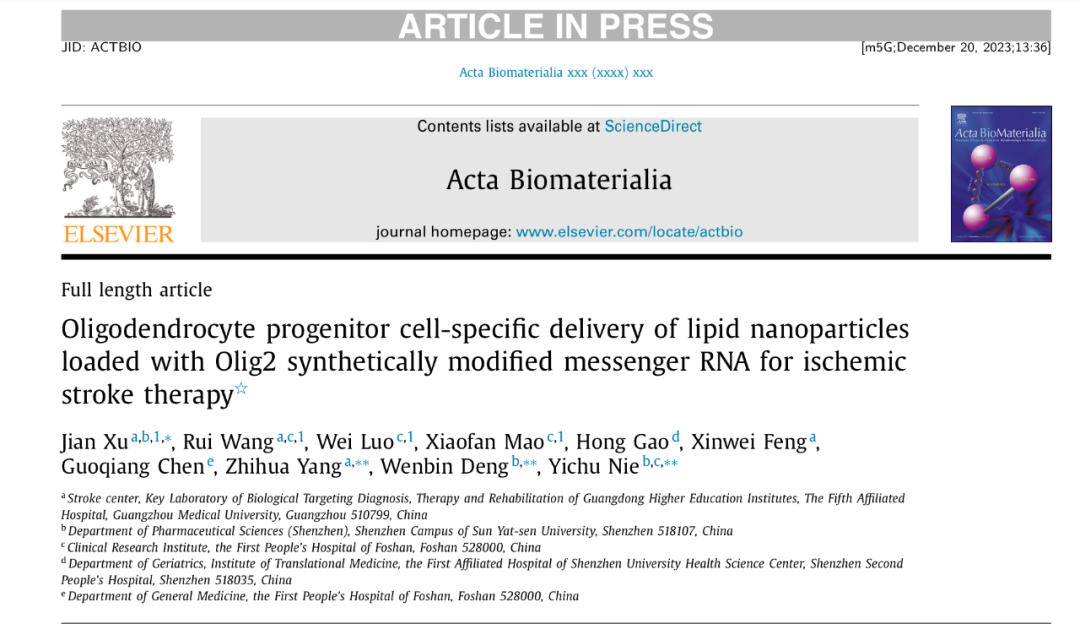The image portrays a website interface, prominently featuring a gray banner at the top with white text that reads "Article in Press." Adjacent to this text, on the right-hand side, the date "December 20th, 2023, 13:36" is displayed. Below this banner, a header states "Contents lists available at Science Direct," flanked by images on either side. The title of the article is "Full-Length Article: Oligodendrocyte Progenitor Cell-Specific Delivery of Lipid Nanoparticles Loaded with Olig-2 Synthetically Modified Messenger RNA for Ischemic Stroke Therapy." This is followed by a list of authors, which appear to be predominantly Chinese names. Further below, there is fine print in black text likely detailing the sources of information, suggesting the study is rooted in Chinese research.